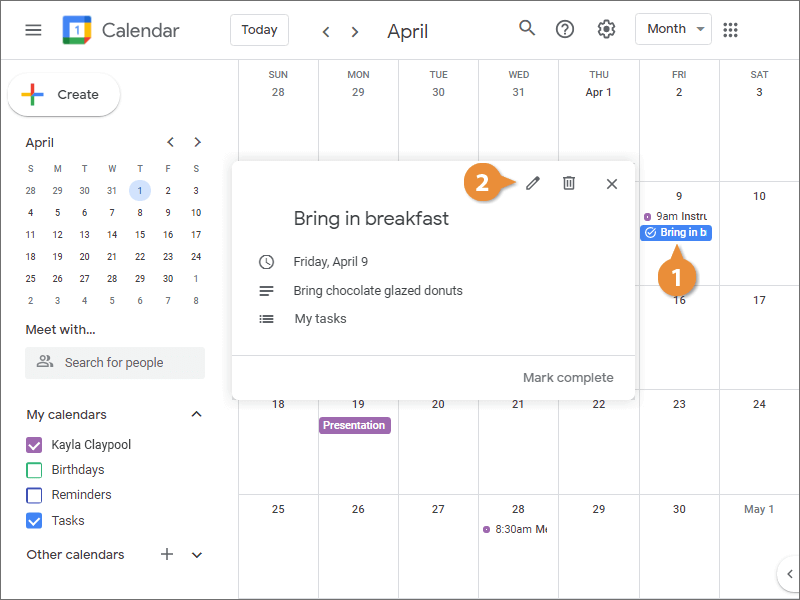In the image, a digital calendar interface is prominently displayed. To the left, it showcases dates for April. The current date, Thursday, April 1st, is highlighted in blue. Below the calendar, there are options to search for people, view "My Calendar" (which is checked), "Bed Days" (unchecked), and "Tasks" (checked), suggesting a customizable view for different categories.

The color scheme within the calendar interface features blue, orange, and green accents, all set against a predominantly white background. Specific dates, such as the 9th, 19th, and 28th, are marked for particular activities. On the 9th, there is a task scheduled. The 19th has a disturbing and inappropriate reminder, which should be corrected immediately as it is highly concerning and unacceptable. Finally, the 28th also has tasks or reminders scheduled.

This detailed setup highlights the user’s organizational approach but also underscores the critical importance of ensuring all scheduled items are appropriate and safe.